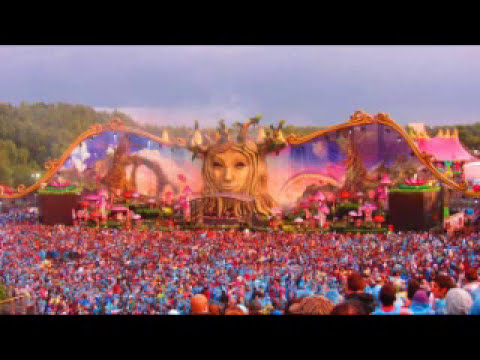The image depicts a large outdoor gathering, possibly at a music festival, with a focus on what appears to be an elaborate concert stage. The crowd, comprising a mix of males and females, predominantly wears blue shirts, creating a sea of blue at the bottom of the image. The stage, placed centrally, features a giant sculpture of a golden woman's head adorned with branches and leaves, resembling Mother Earth. Flanking the stage are mushroom-like structures with brown stems and green tops, adding to the enchanted, whimsical atmosphere. The backdrop of the stage is a colorful, futuristic landscape with hues of pink, purple, and gold, contributing to an almost fantasy-like setting. Trees border either side of the scene, and the sky overhead is cloudy, enhancing the dusky ambiance. The image, though grainy and blurry, vividly captures the vibrant and surreal essence of the gathering, complete with a variety of colors including blue, gray, white, green, orange, purple, and pink.